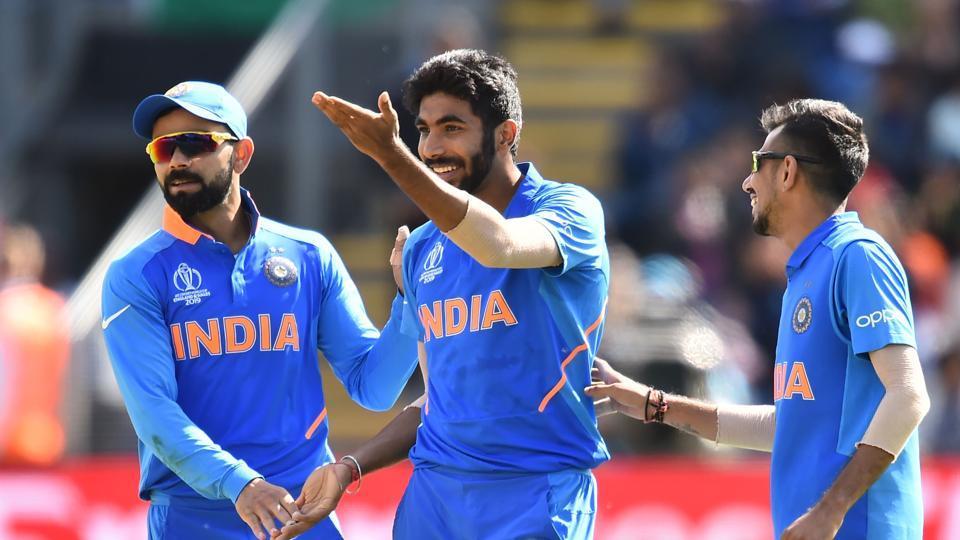In this vibrant, blurred-background photograph, three cheerful Indian men, presumably cricket players, dressed in blue uniforms with the word "India" emblazoned in orange or yellow, are the central focus. The man in the middle, sporting a beard and short hair, raises his left arm with his palm up, seemingly questioning a call. Standing to his left, a man also in a blue uniform dons a matching baseball cap and sunglasses, lightly touching the middle man's shoulder with one hand and his palm with the other, exuding camaraderie. The third man, positioned to the right, is turned slightly sideways, smiling and gently touching the back of the man in the center with his fingertips. All three men are brown-skinned and are clearly enjoying the moment, sharing laughter and high-fives. The red boundary in the stadium and blurred spectators in the background further emphasize the joyful focus on the trio as they celebrate or react to the on-field events.